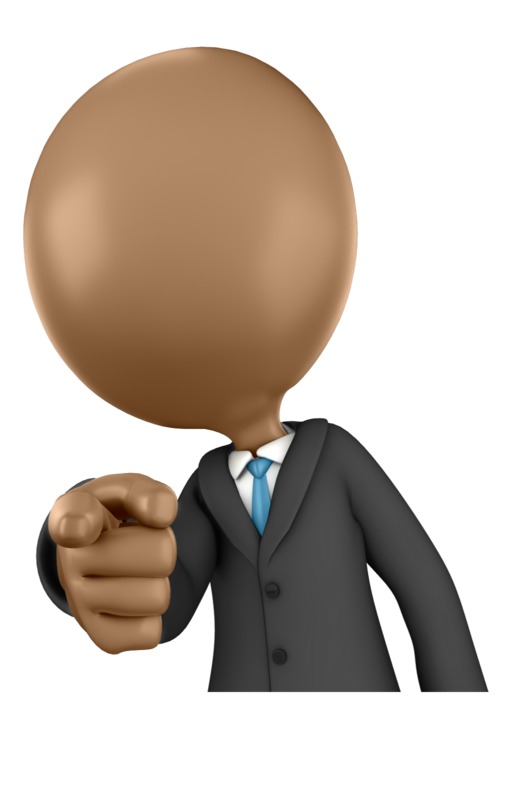The image is a digital drawing of a cartoonish figure that appears to be a person with a large, glossy, balloon-shaped head in a dark brown, tan color. The head lacks any facial features such as eyes, nose, or mouth, and sits atop a very thin neck. The figure is dressed in a black coat, a white business shirt, and a blue tie. This person’s left hand, which is disproportionately large, extends outward, pointing directly at the viewer, while the right arm hangs down. The skin of the hand matches the tan color depicted for the head. The entire drawing is set against a plain, white background. It's a striking and unusual image, somewhat reminiscent of AI-generated artwork due to its odd proportions and peculiar details, such as the misaligned pointing finger.